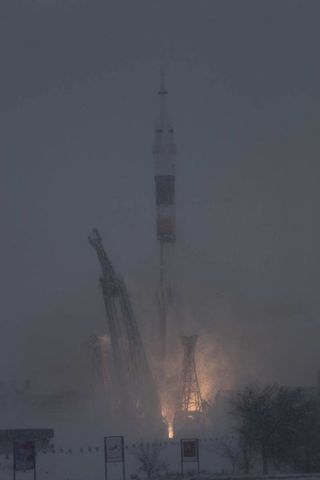The image depicts a foggy, outdoor scene focusing on a rocket about to be launched. The photograph is blurry and low-resolution, making some details indistinct. The rocket itself is a slender, cylindrical structure with a pointed tip, featuring a white body with accents of lighter brown, dark brown, or black, and a line of silver near its top. It rests on a launch pad supported by steel platforms. Below the rocket, flames are visible, indicating the ignition phase with smoke billowing around. In the backdrop, a gray, foggy sky sets a dramatic tone. Surrounding the launch area are signs, including a red and white one and a plain white one, placed along a fence designed to keep people at a safe distance. Trees and bushes are faintly visible through the fog in the lower right corner, adding to the environment's muted, atmospheric quality.